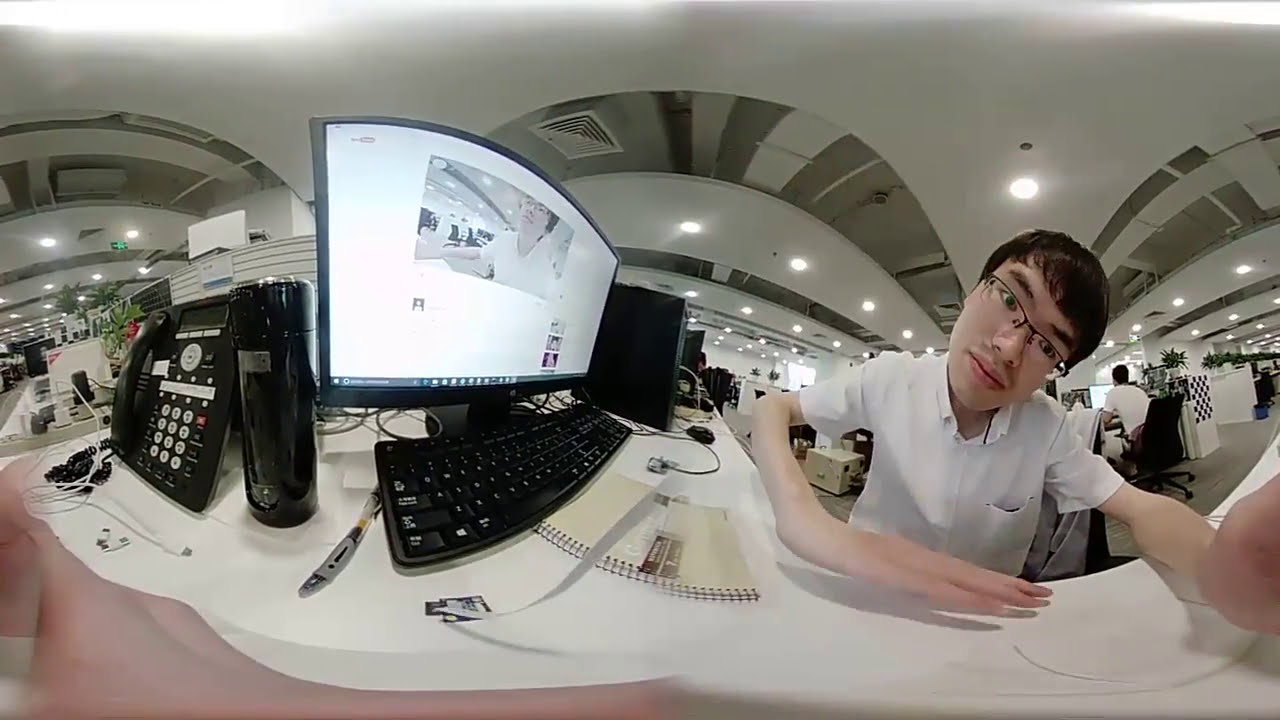The image shows a slightly distorted 360-degree view of a high-end office space, likely located in Japan, characterized by its sleek design and recessed lighting in a white ceiling. Central to the image is a boy with short brown hair, wearing eyeglasses and a white polo shirt. He is seated at a white desk, which contains a black keyboard, monitor, modem, corded phone, and thermos. On the left side of his desk, a computer screen displays a visual related to the camera. The setting suggests a busy, professional environment with multiple workstations, as indicated by the presence of another person seated in a black chair in the room, and various office supplies scattered across the desk. The boy, sporting a playful expression, adds a touch of casualness to the otherwise sophisticated and bustling office backdrop.